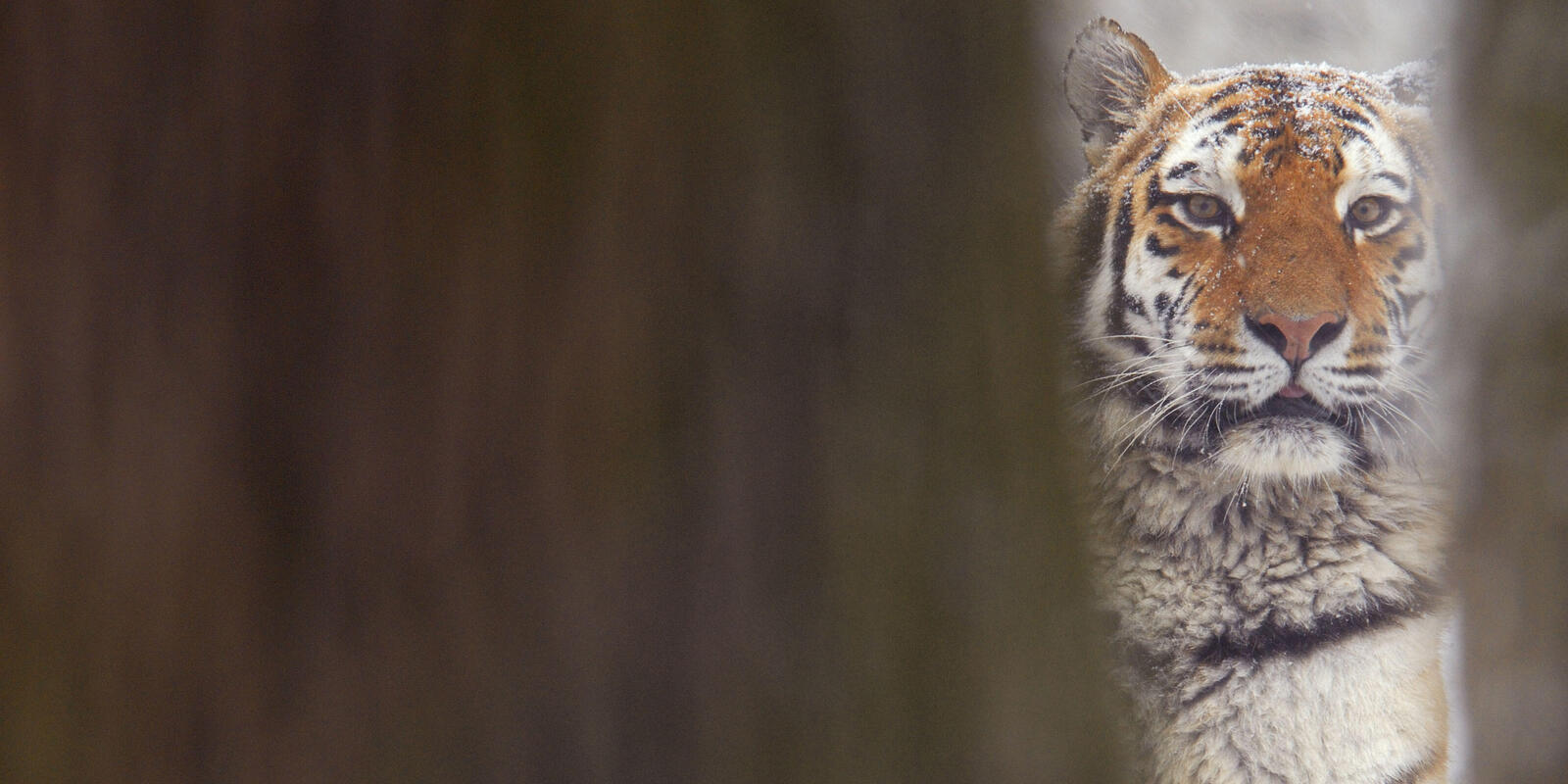This captivating wildlife photograph, rectangular in shape and taken during daylight, features a tiger in a winter setting, with snowflakes visible on its head. The image, about three inches high and six inches wide, prominently features the tiger's head and upper neck peeking out from between two blurred tree trunks. These trunks, with different shades of brown stripes, occupy about two-thirds of the picture from the upper left to the lower right corner, partially obstructing the view.

The tiger stands out sharply in the focus with its intense yellow eyes staring directly at the camera, conveying a powerful presence. Its mouth is slightly open, revealing a pink tongue and white whiskers extending from its cheeks. The tiger's face bears the characteristic orange fur with black stripes, complemented by white patches around its eyes, cheeks, and the thick fur on its chest. One ear is clearly visible, while the other is obscured by a tree.

Overall, the photograph is well-composed, with the blurred foreground enhancing the sharp, detailed focus on the tiger. Despite the potentially intimidating expression of the tiger, it appears calm, unfazed by the presence of the photographer, making it a stunning and intimate glimpse into the natural world.